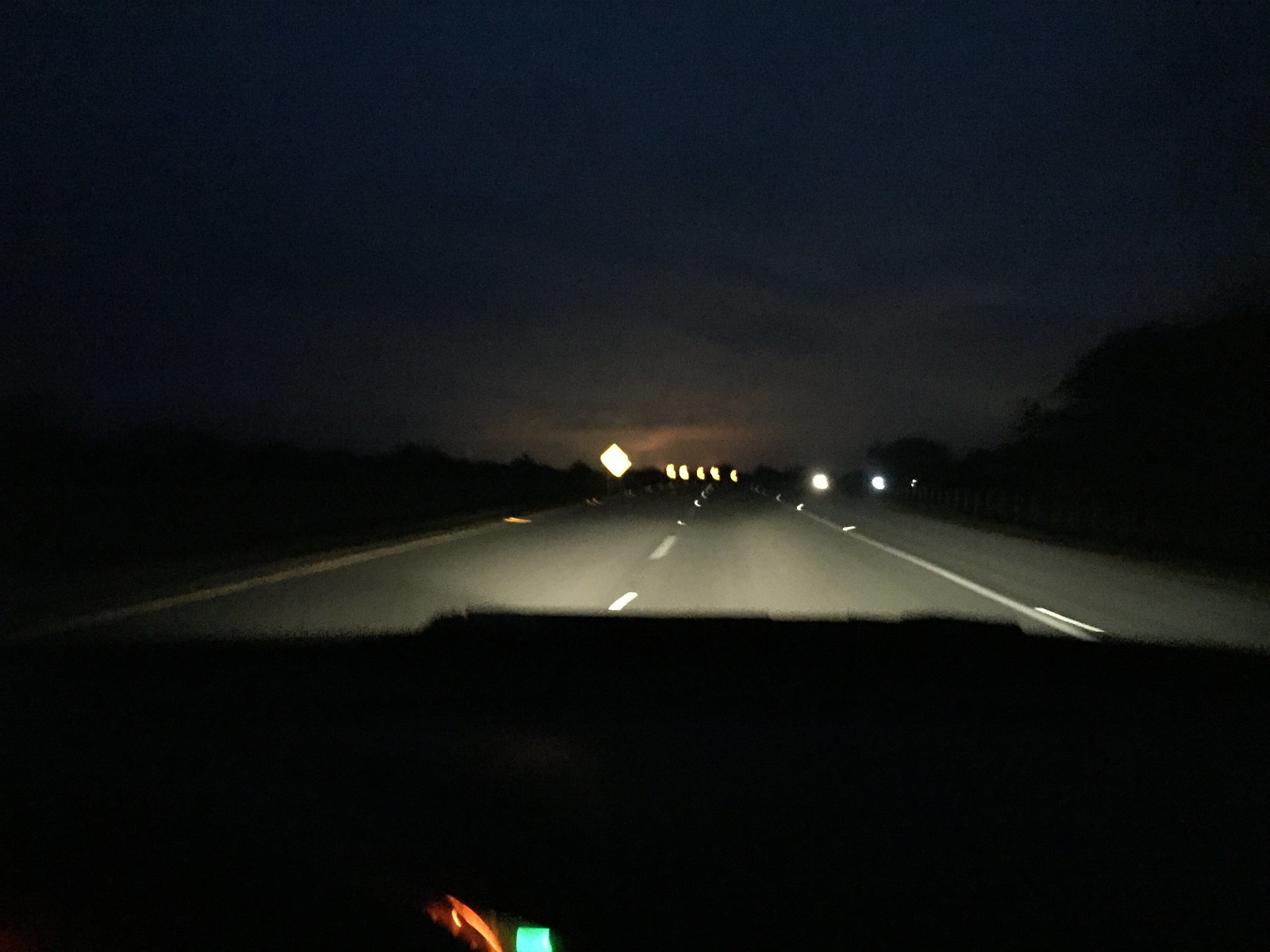The photograph captures a nighttime scene from inside a car, with the dashboard in the foreground and the road stretching out ahead. The sky is a dark gray, almost black, with some textured layers of clouds and a faint, rapidly fading blue light. The road is illuminated by the car's glowing headlights and distant street spotlights, clearly revealing the white lane markings and the concrete asphalt surface. On either side of the road, dark silhouettes of trees are visible, though details are obscured due to the lack of light. Reflective street signs are scattered along the roadside, including a series of yellow caution signs indicating an upcoming curve. In the lower part of the image, parts of the windshield wipers or the car hood create irregular black shapes, and a reflection in the rearview mirror shows a tall green highway sign and an orange object. Additionally, the lane dedicated to emergency pull-offs is faintly visible. Inside the car, the dashboard remains mostly dark, with only hints of red and blue lights from the gauges.